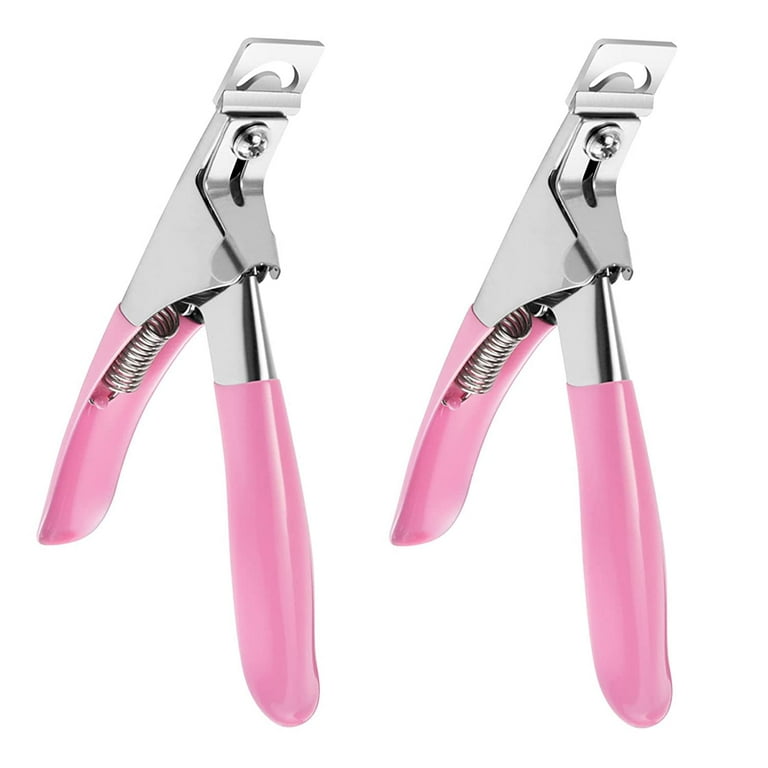This image showcases a close-up of two identical handheld tools, likely nail clippers traditionally used for grooming pets like dogs or cats. The clippers are characterized by their wide, pink rubber handles, designed for a comfortable grip, and a robust, shiny chrome-plated metallic structure. Each tool features a visible spring mechanism nestled under the handle, which allows for responsive, pressure-sensitive operation. There's a small Phillips head screw at the hinge, potentially for maintenance tasks such as tightening, cleaning, or blade replacement. Positioned side by side, they stand on their handles at an angle, with the functional cutting end slightly elevated and the clamping mechanism facing towards the right. The tools appear very new, indicated by their bright and polished finish.